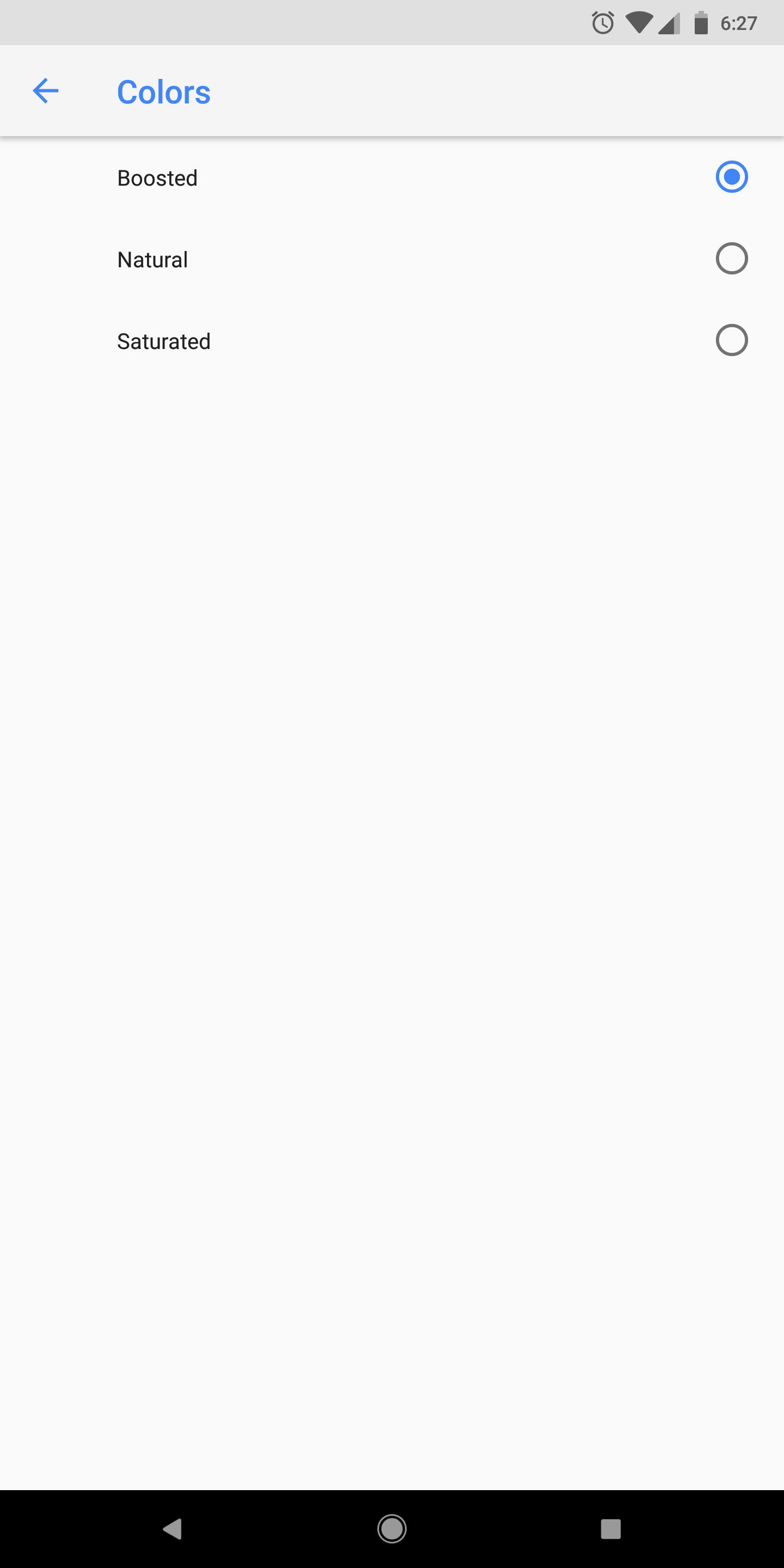This image is a screenshot captured on an Android device. At the top right-hand corner, the time is displayed as 6:27, accompanied by several status indicators: a battery icon, cellular signal bars, a Wi-Fi symbol, and an alarm clock icon. Below these indicators, there is a header featuring a back arrow on the left, with the title "Colors" next to it, both rendered in a blue font.

Further down, the screenshot reveals three display options: "Boosted," "Natural," and "Saturated." Each option has a corresponding radio button on its right, with "Boosted" being the selected choice in this instance. The majority of the screen below these options is blank, displaying a large white space.

At the very bottom of the screenshot, the navigation buttons of the Android device are visible, including the back key, home key, and option key. This layout confirms that the screenshot was taken on an Android phone.